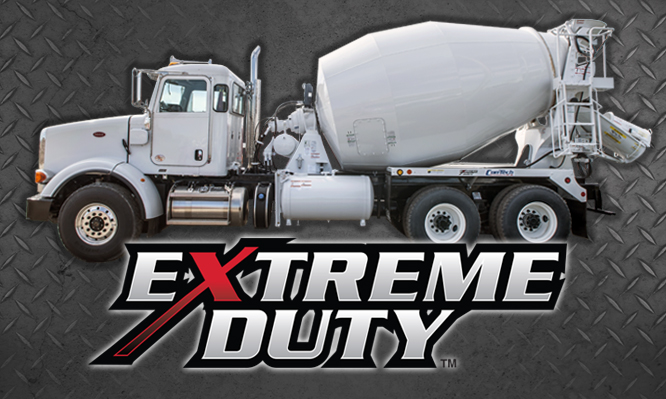The image showcases a white cement mixing truck against a textured black background that mimics tire tracks or metallic steel treads, adding an industrial feel with shades of white and gray. Above the truck, the bold phrase "Extreme Duty™" is prominently displayed, with the X in bright red and the other letters in white, emphasizing strength and resilience. The truck, which is possibly a Peterbilt, is oriented to the left side of the image, allowing a full side view of its three-axle configuration—two in the back with dual tires on each side, totaling eight rear tires, and two front tires. The concrete mixer is visible on the right side of the image, indicative of its functional role. The overall aesthetic is highly detailed and reflective of heavy-duty construction equipment.